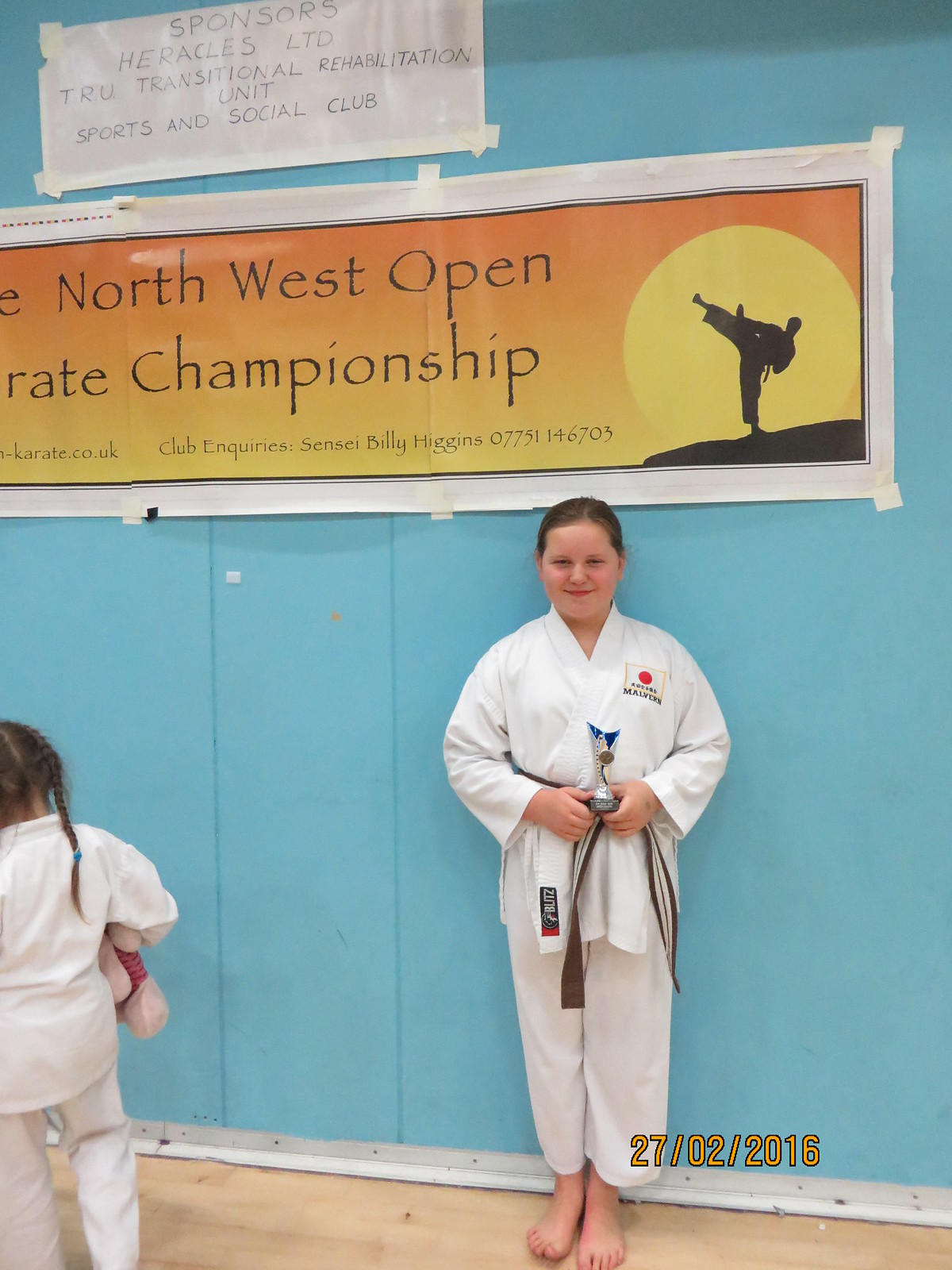This photograph captures a vibrant moment at the Northwest Open Karate Championship, which took place on 27/02/2016. The setting features a padded light blue wall adorned with a prominent banner. The banner, with an orange-to-yellow gradient, displays black text that reads "Northwest Open Karate Championship." It also provides contact information, stating "Club Inquires, Sensei Billy Higgins" along with a phone number. To the right on the banner, a black silhouette of a person performing a karate kick under a yellow sun adds a dynamic visual element.

Front and center stands a young girl of Caucasian descent, likely a teenager, proudly wearing a white karate gi adorned with various patches, including one resembling the flag of Japan on her left shoulder and another with the name "Malvern." She sports a brown belt with horizontal white stripes and smiles while holding a silver and blue trophy. Her eyes meet the camera confidently, capturing her accomplishment and joy.

In the lower left-hand corner, a smaller girl, possibly around seven years old, is visible from the back. She, too, wears a white gi and clutches a stuffed piglet toy, subtly highlighting the younger participants' involvement in the event. A handwritten white paper above with the words "Sponsors, Herakles LTD, True Transitional Rehabilitation Unit, Sports and Social Club" further details the community support for the event. The overall scene is lively and celebratory, embodying the spirit and camaraderie of the karate community.